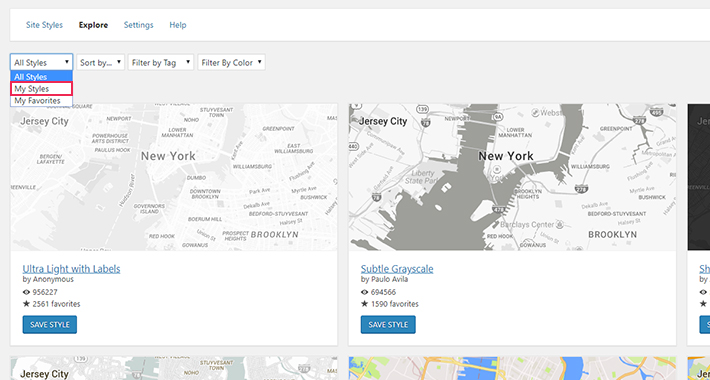Here is a detailed, cleaned-up caption for the image described:

---

This image is a screenshot from an unknown website showcasing different map styles. At the top of the website interface, there is a navigation bar with the following menu options: Site Styles, Explorer, Settings, and Help.

Below the navigation bar, there are four dropdown menus. The first dropdown, labeled "All Styles," has been clicked open to reveal three options: All Styles, My Styles (highlighted in red), and My Favorites. The subsequent dropdowns are labeled "Sort By," "Filter By Tag," and "Filter By Color."

The main content displays two maps detailing the New York and Jersey City areas. The first map is labeled "Ultra Light with Labels" by Anonymous and highlights various neighborhoods and landmarks such as Jersey City, Bergen/Lafayette, Newport, Powerhouse Arts District, Paulus Hook, Lower Manhattan, NoHo, Stuyvesant Town, Governor's Island, the Hudson River, Red Hook, Dumbo, Downtown Brooklyn, Boerum Hill, Brooklyn, Prospect Heights, Bedford-Stuyvesant, Decalto Avenue, Bushwick, Myrtle Avenue, Park Avenue, Flushing Avenue, Williamsburg, East Williamsburg, and Greenpoint. This map has garnered 956,227 views and 2,561 favorites, and it includes a "Save Style" button.

The second map, "Subtle Grayscale" by Paolo Avila, presents the same geographic area but is rendered in a darker, more subdued style. This map has accumulated 694,566 views and 1,590 favorites, and it similarly offers a "Save Style" button beneath it.

---

This caption offers a thorough and structured description of the elements present in the screenshot.